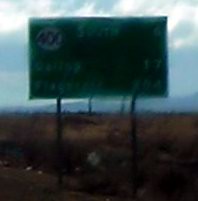The image features a small, blurry photograph depicting a scenic landscape. The bottom half of the image shows a stretch of brownish land, devoid of any distinct details due to the blurriness. Prominently positioned in the scene is a large sign that appears to be mounted about 6-7 feet above the ground. The sign looks quite sizable, estimated to be approximately 6-7 feet high and 10-12 feet wide. There's an indistinct shape, possibly a circle, located at the upper left-hand corner of the sign. The backdrop reveals a sky with a mix of blue hues and gray clouds, suggesting a partly cloudy day. In the distance, there are large, rolling hills that rise from the brown landscape and extend towards the horizon, partially obscured by the bottom of the sign.